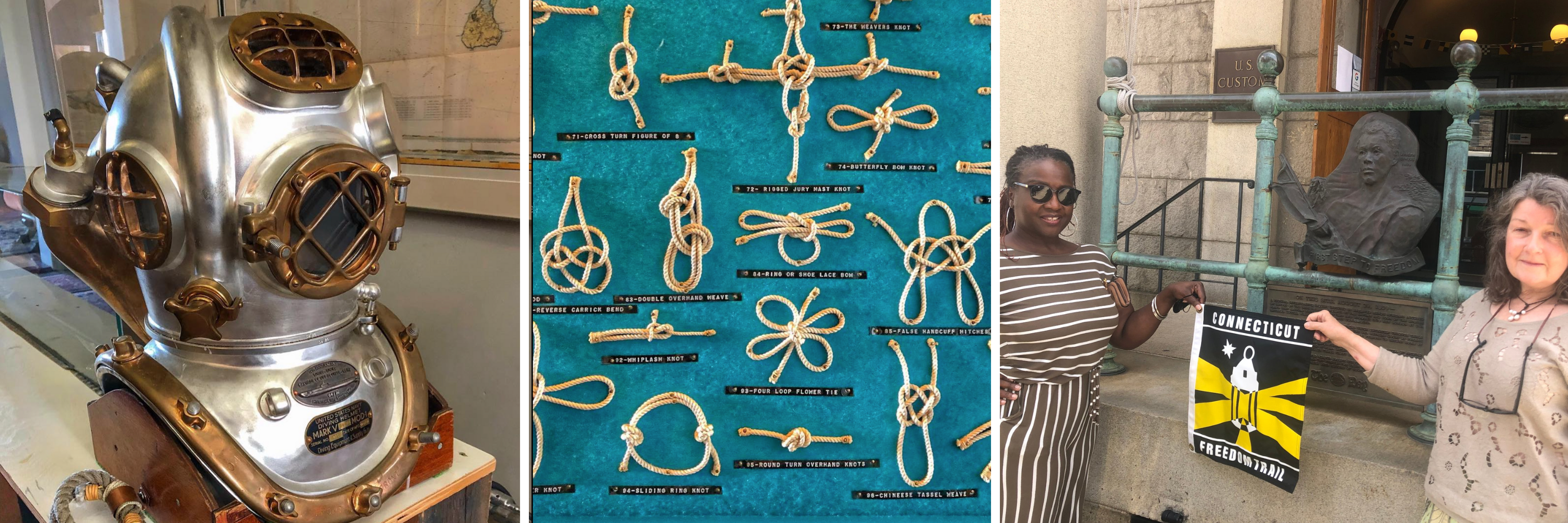The displayed image is a horizontal triptych consisting of three distinct pictures. The first image on the left shows an old-fashioned deep-sea diver's helmet made primarily of metal with gold plating around the face opening, ears, and top of the head. This helmet, sitting on a white table, is set against a backdrop that appears light blue with a white map hanging on the wall behind it.

The central image illustrates various sailor knots against a blue background, with each knot tied using tan-colored rope. Beneath each of the 12 knots is a small description in white text on black backgrounds, though these are not clearly legible.

The final image to the right features two women, one black and one white, standing together and holding a flag that reads "Connecticut Freedom Trail" in white text against a black background, with yellow and white lines. The black woman on the left is wearing black sunglasses and a brown and white striped outfit, while the white woman on the right has gray hair and wears black glasses around her neck and a tan shirt with brown designs. They are positioned in front of a bronze-colored, weathered fence, with a gray ledge and green railings behind them. In the background, a statue mounted on a black brick base is visible, amidst gray and white walls.